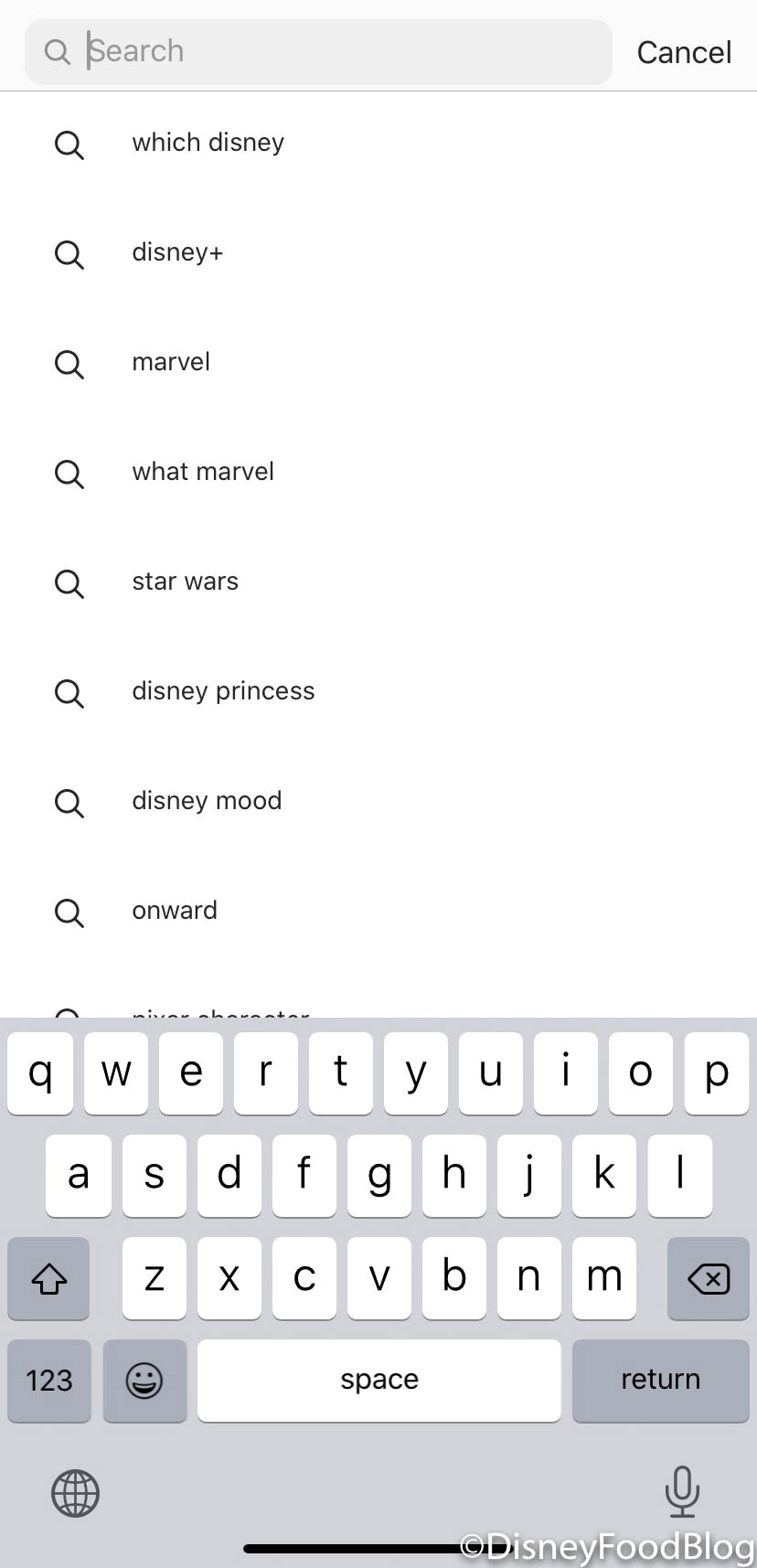This is a cropped screenshot of an iPhone search interface with a white background. At the top, there's a search bar displaying the word "Search" in gray letters. To the right of the search bar, the word "Cancel" is written in black letters. A small horizontal cursor is visible towards the left side of the search bar, indicating that text was being typed. Below the search bar, there is a vertical list of past searches. Each search entry is preceded by a magnifying glass icon. The list includes the following search terms: "which Disney," "Disney plus," "Marvel," "what Marvel," "Star Wars," "Disney princess," "Disney mood," and "onward." The top of another search term is partially visible but obscured by an on-screen keyboard. At the bottom right corner of the screenshot, there is a watermark for Disney Food Blog.